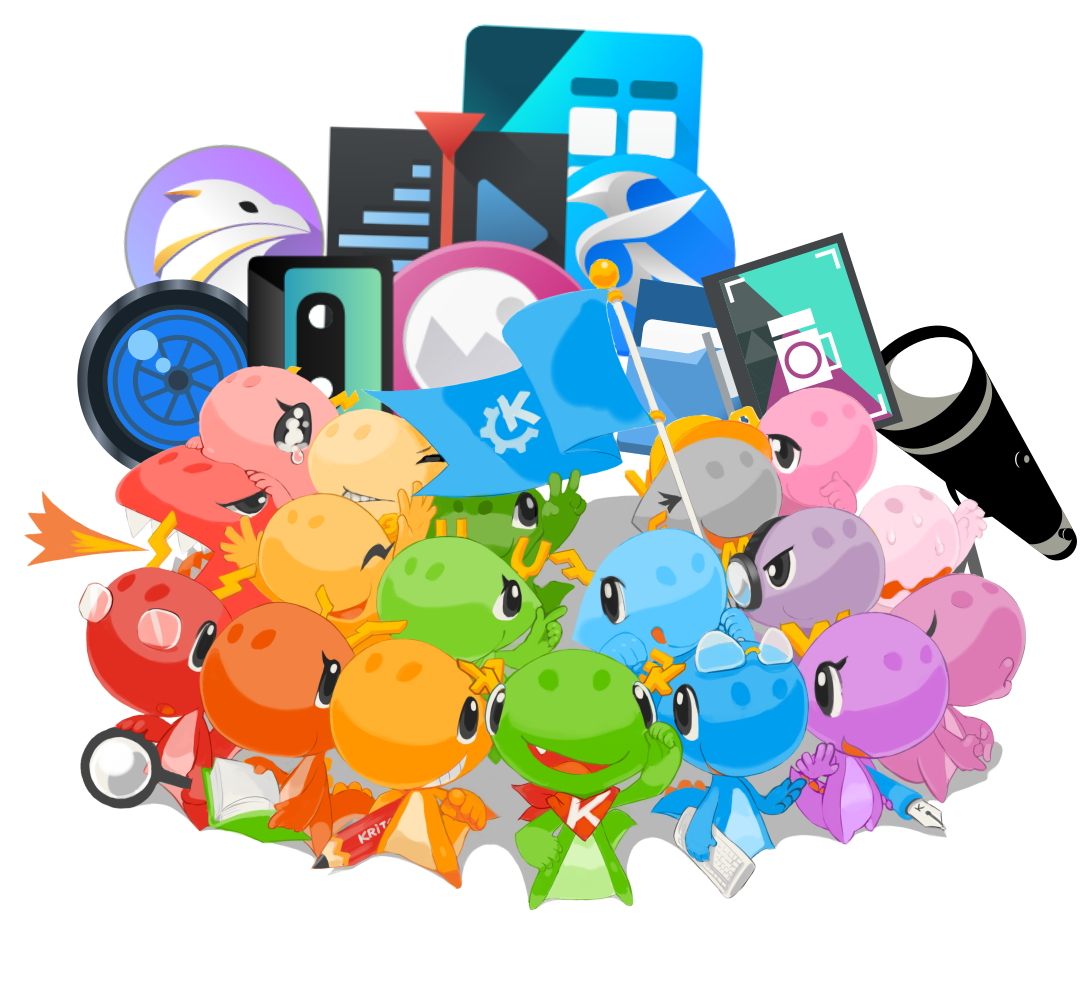This captivating digital illustration brims with vibrant, cohesive elements tailored for the KDE Community, an online hub for software developers, artists, and writers. The central focus of the image features 18 charming, multi-colored characters resembling dragons or dinosaurs, each unique yet harmoniously interwoven. These whimsical creatures are depicted engaging with various tools emblematic of creation and curiosity: papers, pens, magnifying glasses, and more. The backdrop pulsates with dynamic, pictorial-style graphics such as computer screens, cassette tapes, and charts, symbolizing the diverse spectrum of creativity within this community. This artful composition superbly encapsulates the collaborative and innovative spirit of the KDE Community, uniting creators from different realms.